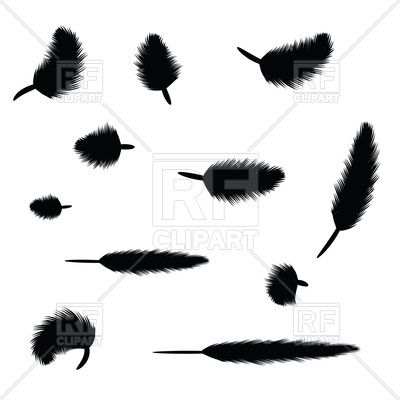The image features 11 black feathers of varying short to medium lengths, positioned at different angles. The feathers populate the screen in an apparently random arrangement with none of them centered. Their positions can be detailed as follows: the upper left feather points at the 1 o'clock position, followed by one at noon, then another around 3 o'clock. Moving down to the next row, the feathers are directed at 9 o'clock, 6 o'clock, and noon respectively. In the subsequent row, a small feather is directed at 9 o'clock, followed by another one pointing at 3 o'clock and one at 9 o'clock. In the last row, one feather arches from the lower right towards the lower left, and the final feather points at 3 o'clock in the lower right. The only colors present are black, white, and gray, all beneath a prominent watermark that reads "RF Clipart," indicating the image is likely sourced from an online clipart website.